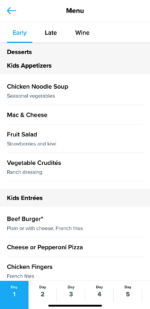This image is a screenshot taken from someone's cell phone displaying a menu page. At the top of the screen, there is a black header with the word "Menu" prominently displayed. In the upper left corner, there is a left-pointing arrow. Below this arrow, the word "Early" is highlighted in blue with a blue line underneath it, while "Late" and "Wine" are listed adjacent to it. 

Under the heading "Early," the menu items are:
- Desserts
- Kids
- Appetizers
- Chicken Noodle Soup
- Steamed Vegetables
- Mac and Cheese
- Fruit Salad
- Strawberries and Kiwi
- Vegetable Crudités with Ranch Dressing

The "Kids" section under the "Early" heading includes:
- Beef Burger (plain or with cheese)
- French Fries
- Cheese or Pepperoni Pizza
- Chicken Fingers with French Fries

At the bottom of the page, five boxes labeled "Day 1," "Day 2," "Day 3," "Day 4," and "Day 5" are present. The "Day 1" box is highlighted in blue, while the remaining boxes are white.